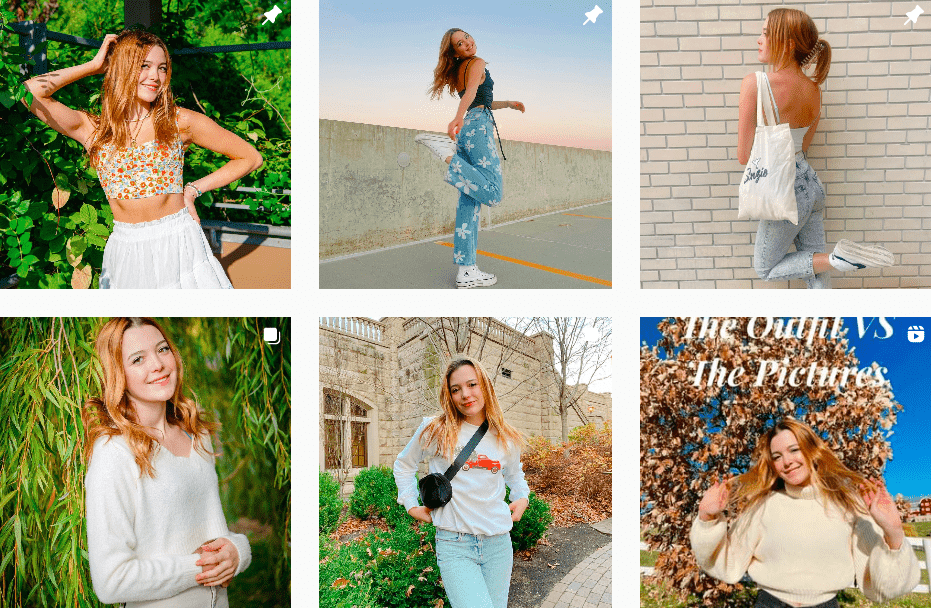The image is a collage of six color photographs featuring the same girl, arranged in two rows of three. In the top left, the girl poses in front of green plants, donning a sleeveless cropped top with orange and blue patterns and a white skirt, her long brown hair flowing naturally. In the top middle, she stands with her back to the camera, glancing over her shoulder, wearing blue jeans adorned with white flower patterns, white socks, white shoes, and a black tank top. The top right shows her from behind with one leg lifted, dressed in blue jeans, a white top, and carrying a white shoulder bag.

The bottom row continues to showcase her versatility. The bottom left photograph features her in a white cardigan over a white top, and she's positioned similarly in the middle bottom image, this time in a white sweatshirt with blue jeans and a crossbody bag, standing in front of what appears to be an institutional building in autumn. The bottom right image captures her holding her hair with both hands, posed in front of a brown tree, wearing a white sweater with the title "the outfit versus the picture" above her. This detailed, cohesive portrayal underscores the girl's diverse fashion choices and varied backdrops, aligning with themes of fashion photography and representational realism.